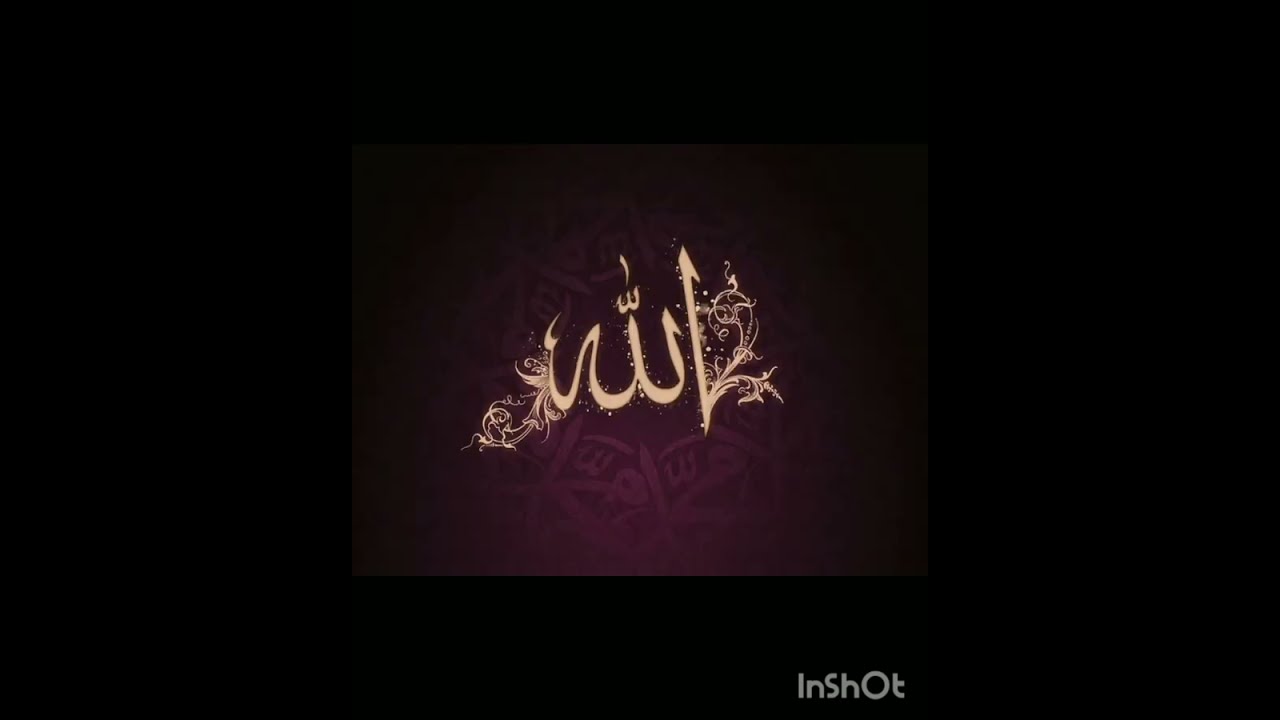The image appears to be a highly stylized digital screenshot, possibly resembling an album cover or an advertisement. The backdrop is predominantly black with intricate dark purple designs and patterns. Central to the image is a sophisticated gold emblem that features a fanciful, detailed "W." This "W" is uniquely designed, with an extra hump and adorned with elegant flourishes that resemble plant life, including flowers, leaves, and curling tendrils. To the right of this emblem, there is a sharp, straight line with a pointed tip, also embellished with floral elements branching off and curling around it. The emblem gives off a sense of sparks and fairy dust, adding to its ethereal aesthetic. At the bottom right corner, the word "InShot" is prominently displayed in gold, set against the dark purple background.

This composite description captures the shared and emphasized elements from the three voice captions, providing a detailed and cohesive portrayal of the image.